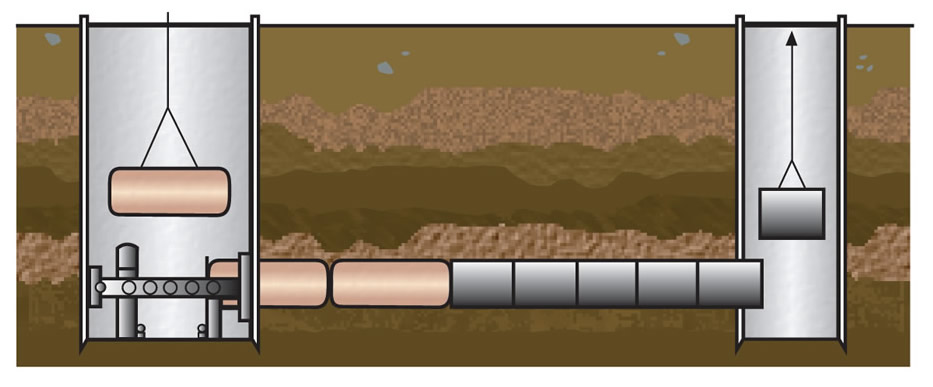The image depicts a cartoonish schematic of an industrial machinery system embedded in the ground, with visible layers of earth in the background shaded in different tones of brown and gold. The drawing features two vertical cylindrical shafts on each side, connected by a horizontal tube or mechanism. In the left shaft, a solid, oval-shaped object is being lowered toward a mechanism below, while on the right shaft, a square, silver object is being pushed upward, as indicated by arrows. The machinery resembles an industrial or factory assembly-line process. There's a hook and possibly a conveyor belt involved, with various components depicted in shades of gray, pink, gold, and silver, though there are no textual labels or annotations on the image.